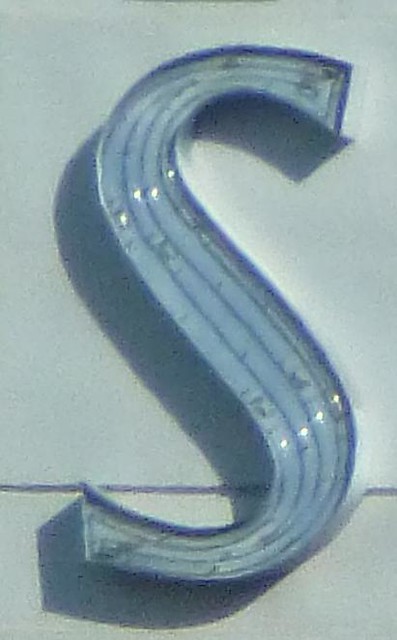This photograph presents a closely zoomed-in, slightly grainy image of the letter 'S,' which appears to be crafted from metal. The metallic 'S' is affixed to a predominantly white surface, with a dark, thin dividing line running horizontally near the bottom. This line segregates the background into two segments: the upper larger white area and a smaller, slightly darker section at the bottom. Adorning the 'S' are eight small lights, positioned symmetrically with four lights accentuating the lower curve and the remaining four illuminating the upper curve, contributing a subtle glow to the overall metallic finish.